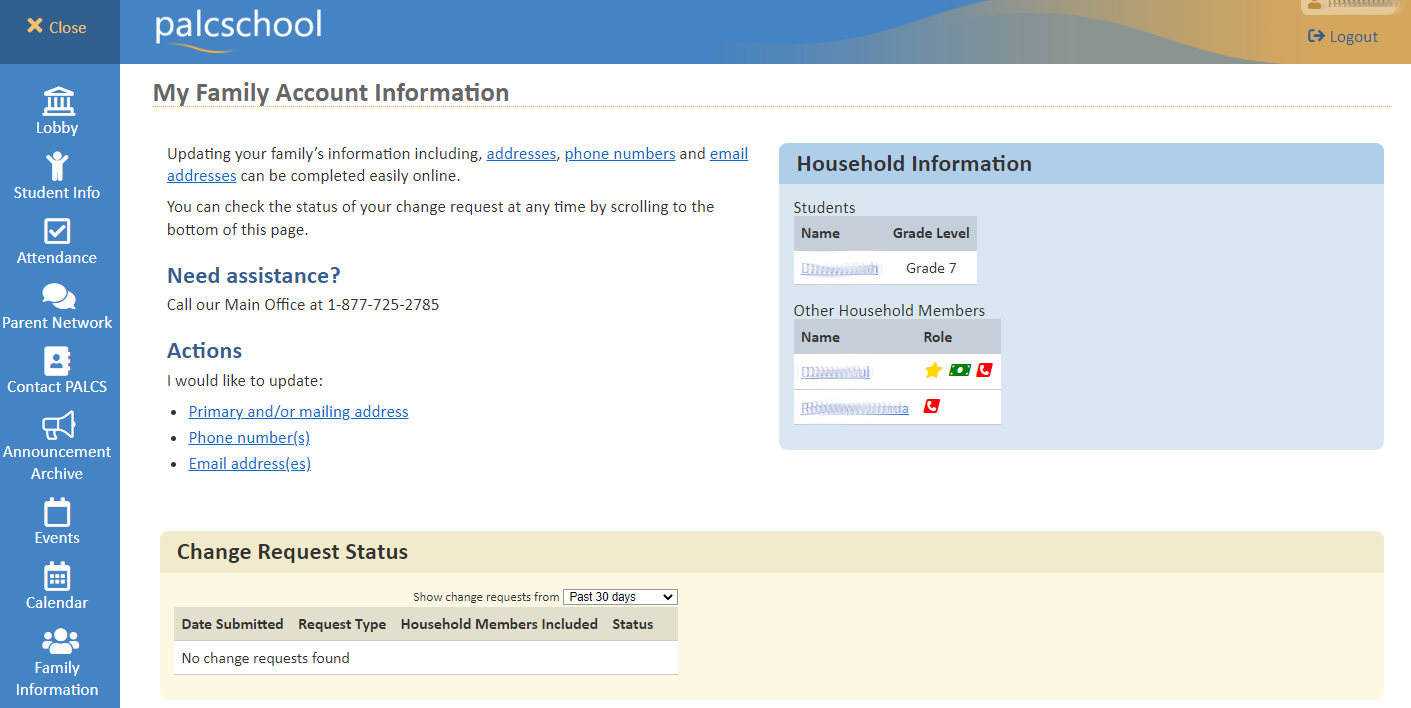The screenshot displays a web page with a clean, white background, specifically from the PLACS school system. The page includes several headers and sections organized as follows:

1. **Top Navigation Bar:**
   - Close
   - Lobby
   - Student Info
   - Attendance
   - Parent Network
   - Contact
   - PLACS (PA Leadership Charter School)
   - Announcement
   - Archive
   - Events
   - Calendar
   - Family Information

2. **Main Content:**
   - **Updating Your Family's Information**
     - This section emphasizes the importance of keeping family information up to date.
     - It informs users that they can easily update their family's information, such as addresses, phone numbers, and email addresses, online.
     - The links to update addresses, phone numbers, and email addresses are highlighted in blue for easy access.
     - Users can also check the status of their change requests at any time by scrolling to the bottom of the page.

3. **Assistance Information:**
   - There is a note in blue text instructing users to call the main office at 1-877-725-2785 if they need assistance.

4. **Actionable Links:**
   - Below the assistance note, there are three hyperlinks labeled "I would like to update":
     - **Primary and/or Mailing Address**
     - **Phone Numbers**
     - **Email Addresses**

Each of these links allows users to update specific types of contact information, making the process straightforward and user-friendly.